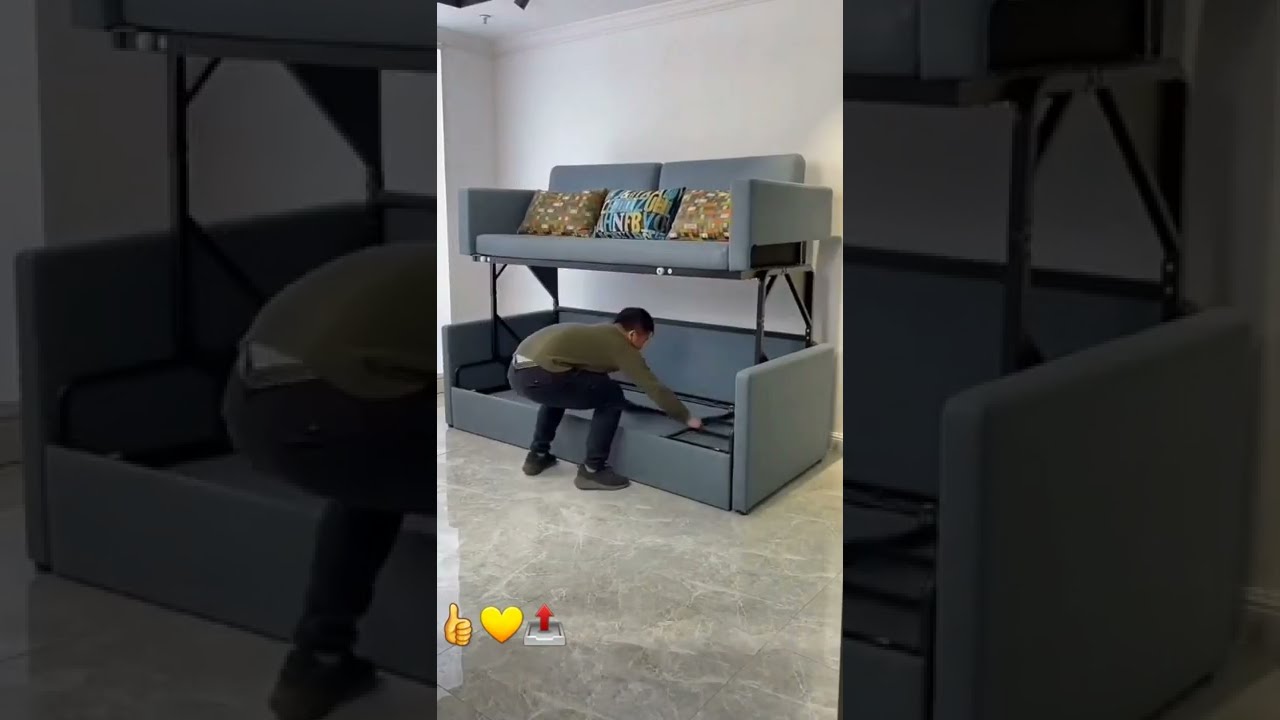This horizontal rectangular image presents a complex scene centered around a man manipulating a multi-functional grey sofa. The primary focus, located in the vertical center, features a man dressed in an olive-green long-sleeve top, black pants, and black shoes. He is bent over in a flat-back position, working with the internal frame of the sofa, which appears to be a two-tier, bunk bed-style unit. The man is either pulling out or putting away the bottom section of the sofa, which is elevated on four legs, revealing a detailed frame beneath. The grey sofa has a matching upper section adorned with three throw pillows, set against the white walls and light grey marbled tile floor of the room. Enhancing the composition, the lateral thirds of the image offer black-and-white, slightly blurred close-ups of the sofa, creating a repetitive, dim background. Additionally, three icons—a gold thumbs-up, a yellow heart, and a red upward arrow—are positioned at the lower part of the image, adding a digital touch.